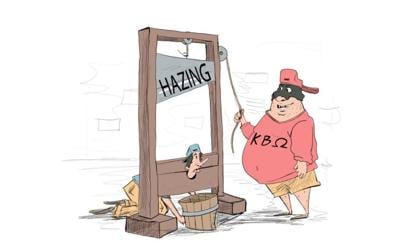This hand-drawn cartoon illustrates a stark message about hazing in fraternities. On the right side of the image, a large, overweight man with a large belly wears a pink sweater emblazoned with "KB Omega" along with the Omega symbol. He also sports a pink baseball cap worn backwards, yellow shorts, and a black mask over his eyes. He is depicted holding the rope of a massive wooden guillotine, poised to drop its sharp blade. The blade has "hazing" inscribed across it. Beneath the blade, a much thinner individual has their head positioned in the guillotine, wearing a blue baseball cap and a blue shirt with yellow pants visible behind the wooden frame. A bucket is strategically placed beneath the guillotine to catch the head when the blade falls. The background is primarily white, with subtle grey lines suggesting the dimensions of a floor and a brick wall behind them, emphasizing the severity and isolation of the scene. This cartoon powerfully critiques hazing practices within fraternities, suggesting a call for its end.